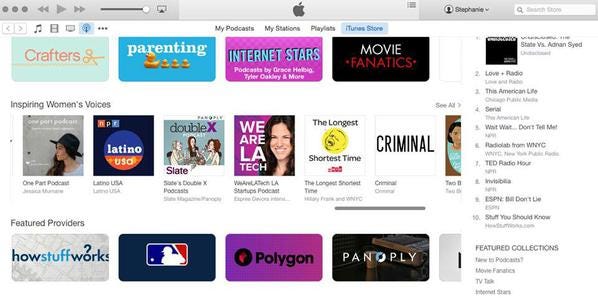The image is a screenshot of the Apple iTunes Store, showcasing a variety of entertainment options available for users. At the top of the page, there are several categories listed, including "Crafters," "My Stations," "Playlists," and "iTunes Store," with the latter highlighted, indicating that the current view is of the iTunes Store section.

The first image on display is categorized under "Crafters," followed by sections labeled "Parenting," "Internet Stars," and "Movie Fanatics." Below these categories, there is a segment titled "Inspiring Women's Voices." This section highlights podcasts such as "Latino USA," "Double X," "We Are LA Tech," "The Longest Shortest Time," "Criminal," and another title that is partially cut off from view.

Further down, the "Featured Providers" area is displayed, including content from "How Stuff Works," "Major League Baseball," "Polygon," and "Panoply." 

On the right-hand side of the image, there is a vertical list that begins with "State vs. Aaron Syed," followed by "Love and Radio," which appear to be personal recommendations or preferences, although this section lacks a specific header. 

Toward the bottom of the screenshot, there is a section labeled "Featured Collections," which includes various collections and some options with dropdown menus. The text in some areas is very small, making it hard to read.